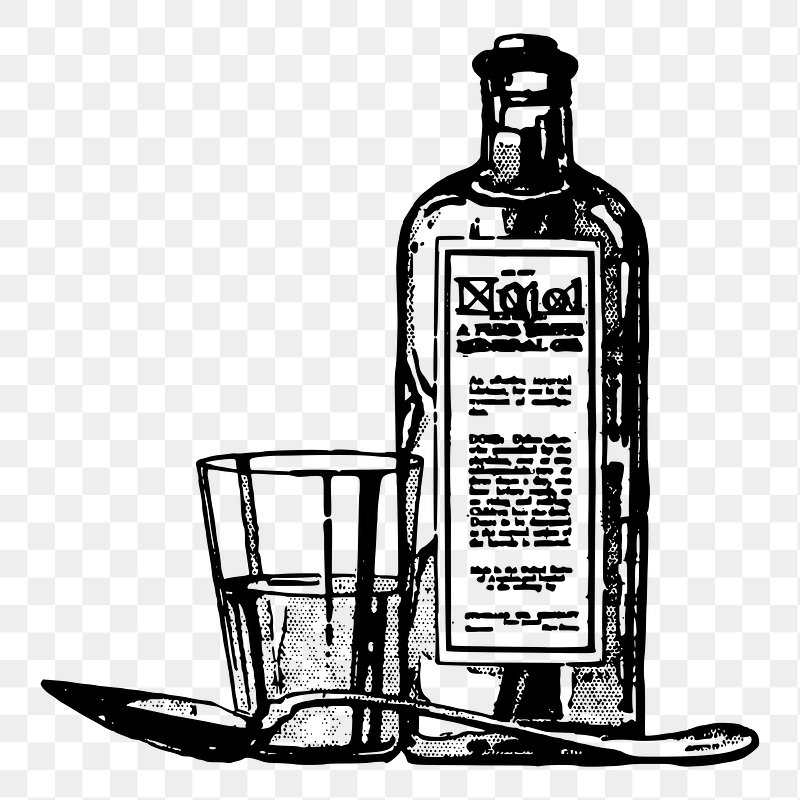This black-and-white image features a hand-drawn, clipart-like illustration on a checkerboard background of muted gray and white tones, often indicative of a transparent background. The scene comprises three main objects: a large, corked bottle with a label on it, a half-full glass tumbler, and an old-fashioned teaspoon placed in front of them. The bottle, possibly a medicine or liquor bottle, has a flattened shape with rounded shoulders. Its label is deliberately illegible, enhancing the clipart's stylized nature. The glass tumbler contains a liquid that's depicted with black polka dots, suggesting a textured or patterned content. The teaspoon, positioned in front of both the bottle and the glass, complements the overall composition with its vintage appearance.